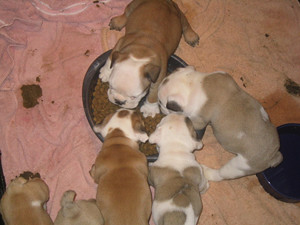In this overhead photograph, a group of seven or eight puppy dogs, mostly with brown and white fur and some with gray and white, are gathered around a large black food bowl filled with dry dog kibble. Four of the puppies are eagerly eating from the bowl, while two stand nearby, seemingly waiting for their turn. The puppies, which appear to be bulldog types, display a mix of color patterns, including a dark brown puppy with a white face and paw, and lighter tan ones with white faces. The setting is a floor covered with dirty pink towels, partially stained with what might be poop. A black water bowl is also visible at the bottom right of the image, and the scene is framed with a sense of playful chaos as the puppies feed.